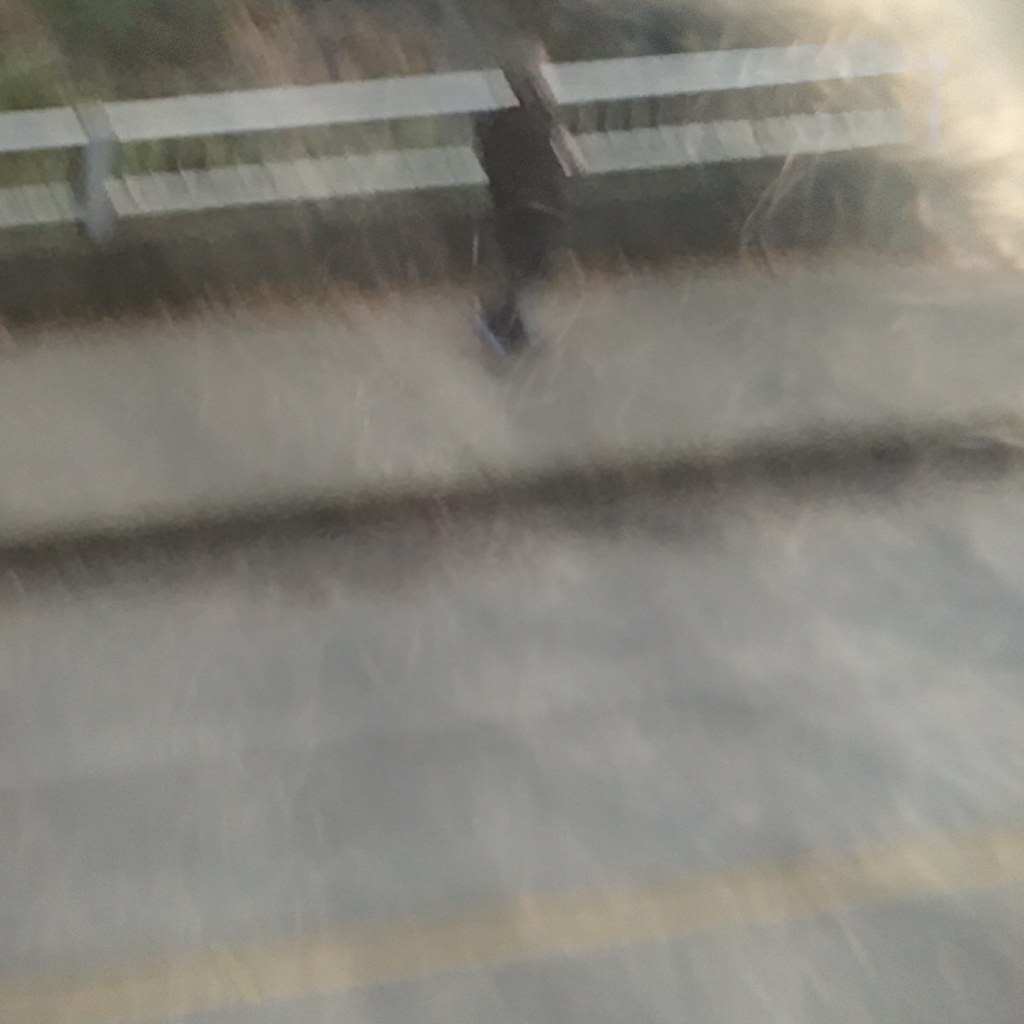The image is a very blurry depiction, resembling a photograph that someone has painted over with a swirling motion. It shows a gray roadway with a visible yellow line, suggestive of a typical road marking. To the side, there is a gray sidewalk where a small boy or perhaps a man is either walking or running. This figure is dressed in darker pants, black and white tennis shoes, and a black and gray sweater or outfit. The face of the figure is light gray and devoid of any distinguishable features, likely due to the blurriness.

Behind the figure is a silver-white metal fence, characterized by two parallel bars that extend from the left side and possibly beyond the bright light source in the upper right corner of the image. The background showcases indistinct greens and beiges, giving it a camouflage-like appearance, with no discernible objects. The entire image is marred by light cream-colored artifacts that resemble scratches or embers, contributing to its overall obscurity and suggesting it might have been manipulated digitally or affected by some form of interference.